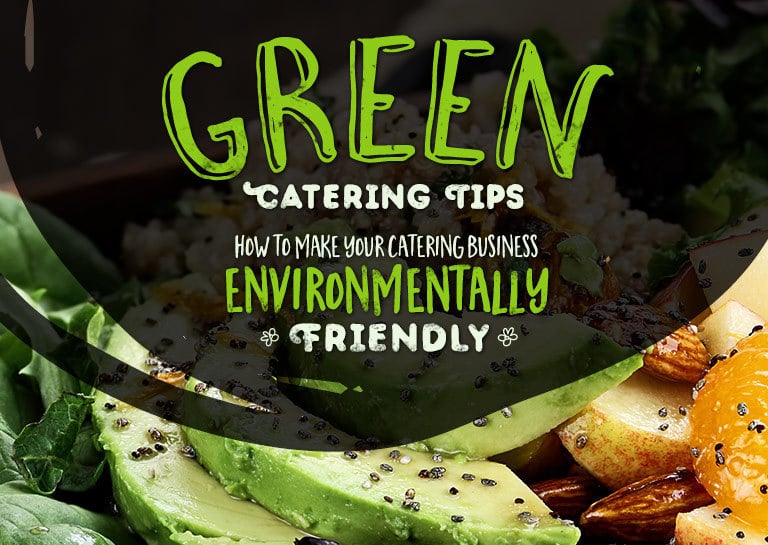This image appears to be a flyer or brochure offering tips on making a catering business environmentally friendly, possibly targeted at green-minded entrepreneurs. The title "Green Catering Tips" is prominently displayed at the top in large, green letters, followed by a subtitle in smaller alternating green and white text that reads, "How to Make Your Catering Business Environmentally Friendly." The word "friendly" is accented with two stylized flower designs flanking it.

The background features a translucent, shadowed half-circle overlay, giving the text a clear backdrop. Behind this overlay, the bottom half of the image reveals a vibrant assortment of fruits and vegetables. Visible items include leafy greens on the left, avocado slices sprinkled with sesame or chia seeds, and a variety of fruit slices such as apples and oranges. Additionally, there are nuts like pecans or almonds, all adorned with a glossy glaze and more black seeds scattered across the display. This vivid arrangement, coupled with the informative text, makes for a visually appealing and educational advertisement about sustainable catering practices.